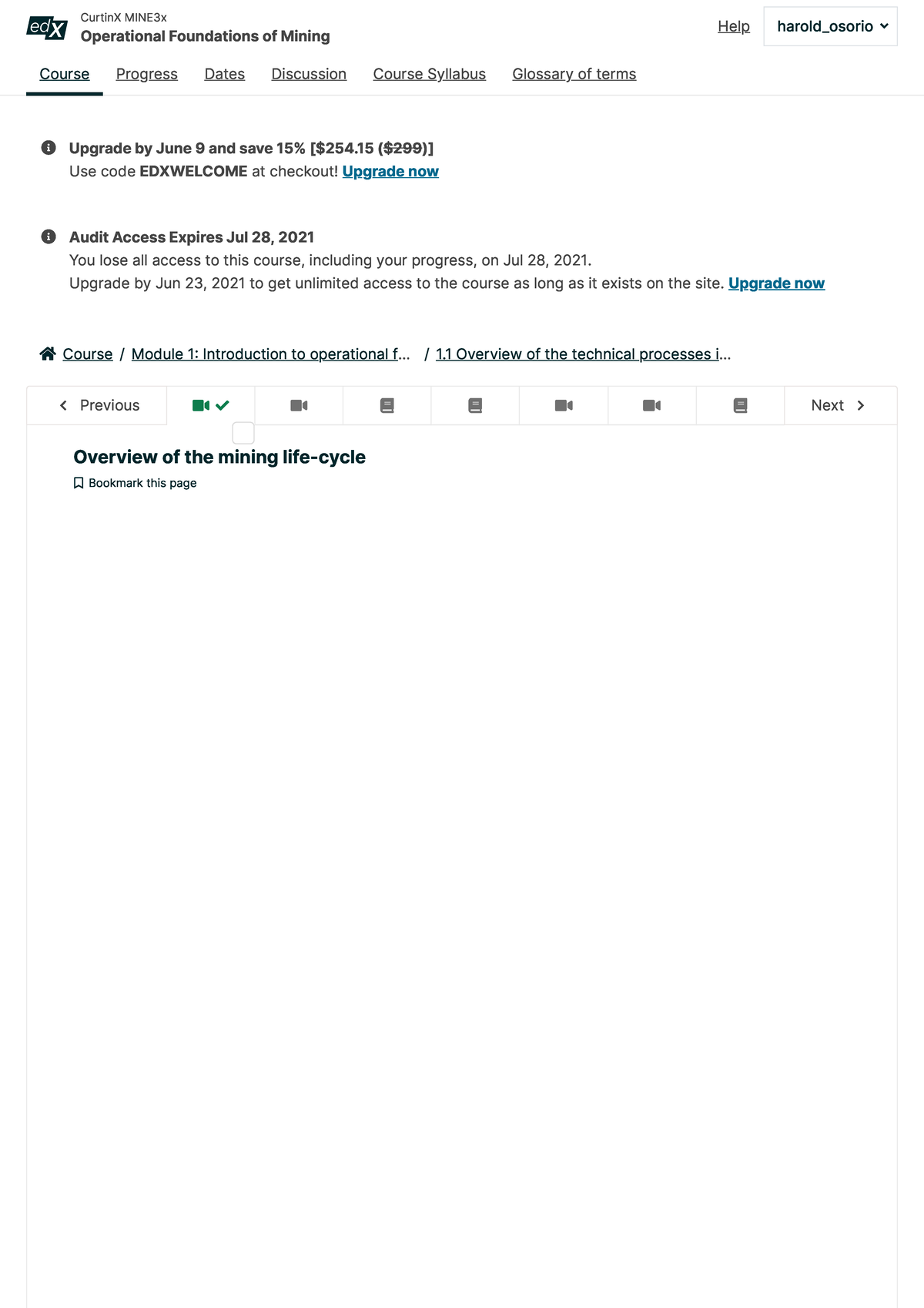This is a detailed and cleaned-up caption for the given image description:

---

The image is a screenshot of a webpage with a minimalistic, white background design. In the upper left-hand corner, the text "Cure Mine 3X" appears prominently, followed by "Operational Foundations of Mining" written in black font beneath it. On the left side, there is a logo consisting of two interlocking squares. The left square has the letters "ED" in white font, while the right square has a white "X," both set against a greenish-gray background.

The webpage seems to be an online course platform, evidenced by the navigation menu at the top. The menu items from left to right are: Course, Progress, Dates, Discussion, Course Syllabus, and Glossary of Terms. Below this menu, a banner headline reads "Upgrade by June 9 and Save 15%." The original price of $299.00 has a line through it, with a discounted price of $254.15 displayed next to it.

---

This caption aims to provide a clear, structured, and detailed description of the website screenshot.